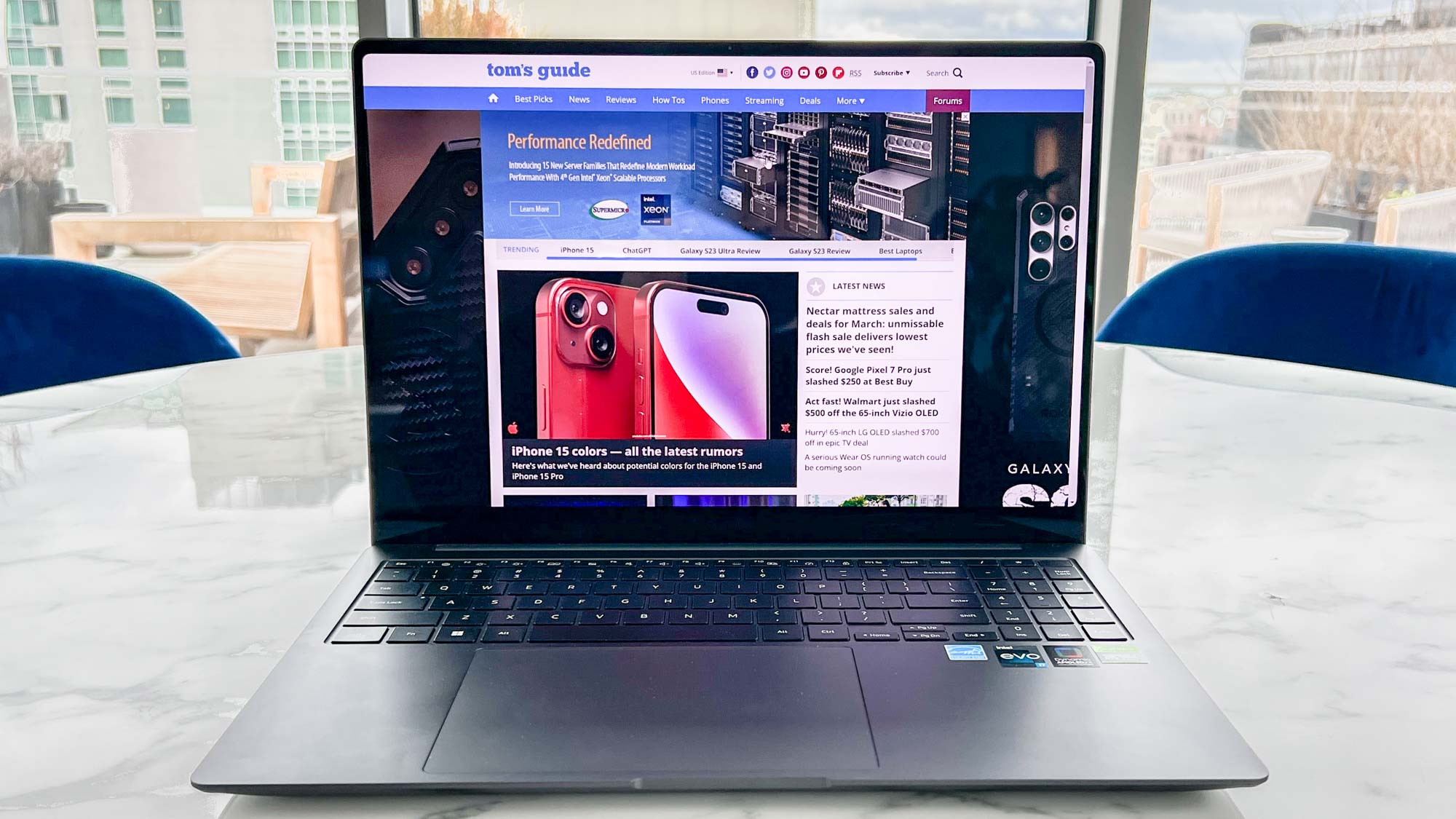The photograph, captured in landscape mode, presents a detailed scene of a black laptop positioned on a reflective, circular white marble table, accompanied by dark blue cushioned chairs on either side. The table appears to be part of a conference room that overlooks a cityscape through three large window panes also visible in the background. The laptop screen displays the homepage of a tech website called "Tom's Guide." The webpage features a range of menu options such as Best Picks, News, Reviews, How-To's, Phone Streaming, Deals, and a prominent red square labeled 'Forum.' Central to the webpage is an article titled "iPhone 15 colors, all the latest rumors," accompanied by striking images of red iPhones, showcasing both their front and back views. The distinctive keyboard of the laptop includes multiple stickers, one of which reads "EVO." The ambient light, ample reflections of the table, and surrounding elements create a professional and vibrant atmosphere.